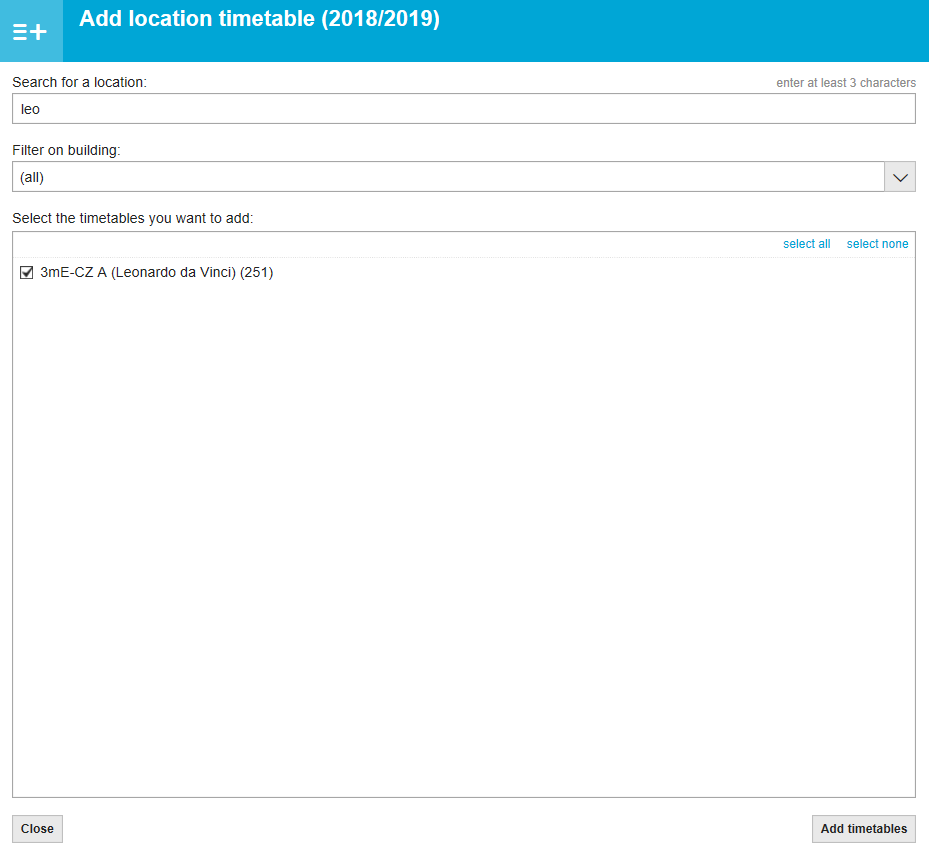The screenshot displays a web interface for adding a location timetable for the academic year 2018-2019. The interface features a blue header bar at the top with the title "Add Location Timetable (2018-2019)." On the left side of the header bar is a small blue square containing three vertical lines and a plus sign next to it.

Below the header bar, the background is all white, featuring three main information fields. The first field, labeled "Search for a Location," includes a prompt at the end of the row that states, "Enter at least three characters." The search field contains the text "LEO." 

The second field, titled "Filter on Building," includes an entry window with a drop-down menu on the far right. The field is populated with the word "All" in parentheses. 

The third field, significantly larger than the others, is labeled "Select the timetables you want to add." Inside this field, on the top-right corner, are two selectable options in blue text: "Select All" and "Select None." On the left side of this window is a single line of information starting with a checked checkbox. This line reads "3M-E-CZ-A (Leonardo da Vinci) (251)."

At the very bottom of the screen are two buttons for further action. On the left is a small "Close" button, and on the right is a wider button labeled "Add Timetables."